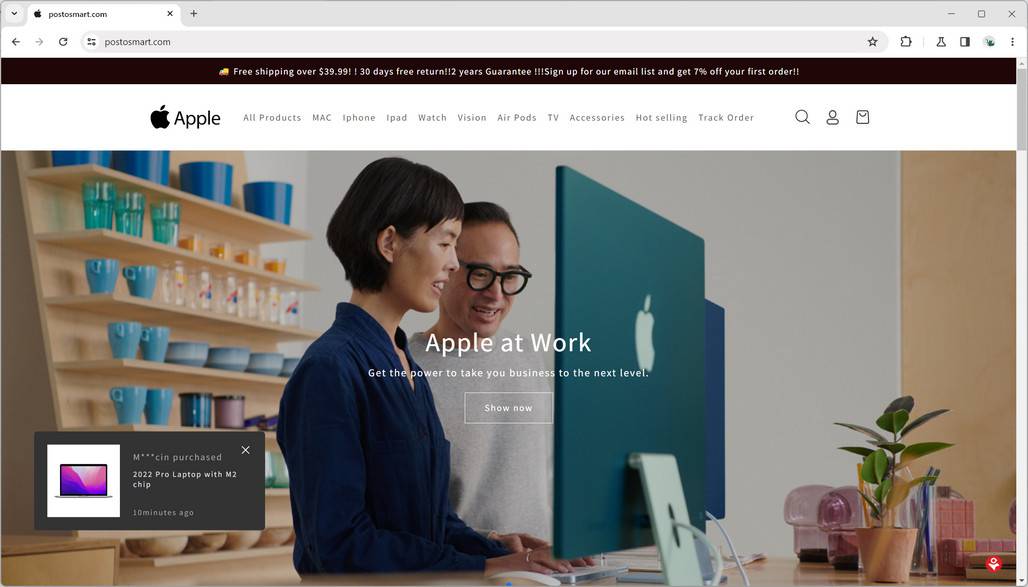The promotional image from Smart.com highlights several key offers: free shipping on orders over $39.99, a 30-day free return policy, and a two-year guarantee on products. It also encourages users to sign up for their email newsletter to receive a 7% discount on their first order.

The advertisement prominently features the Apple logo with the word "Apple" and provides a list of categories including Mac, iPhone, iPad, Watch, Vision, AirPods, TV, Accessories, Hot Selling, and Track Order.

The accompanying picture showcases an "Apple at Work" theme. It depicts two Asian individuals standing in front of iMacs. The man is wearing glasses and a gray sweatshirt, while the woman is dressed in a blue dress shirt. A caption in the image reads: "Get the power to take your business to the next level. Shop now."

In the background, shelves filled with mugs, bowls, and glasses suggest that these individuals may be utilizing Apple products for their business. Additionally, the image indicates that a customer purchased a 2022 MacBook Pro with an M2 chip 10 minutes ago, although the name of the customer is blocked out.